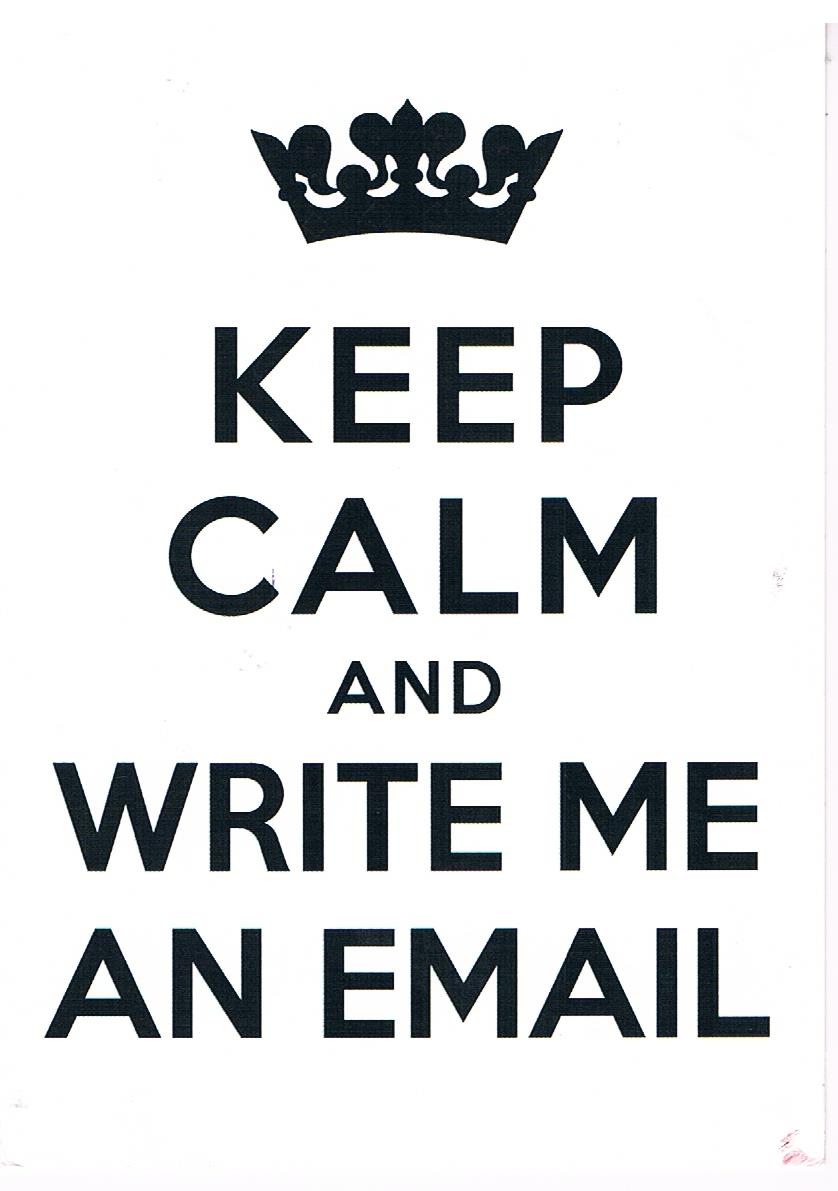The image is a vertical rectangle styled as an internet meme inspired by the famous British wartime poster "Keep Calm and Carry On." It features a white background with centered black ink text. At the top, there is a black and white illustration of a crown with three pointy and four rounded parts. Below the crown, the text reads in plain, all capital letters: "KEEP CALM AND WRITE ME AN EMAIL," distributed over five centered lines. There is also a faint gray or beige band on the right side, suggesting the image might be a scanned copy of a printed sheet of paper.